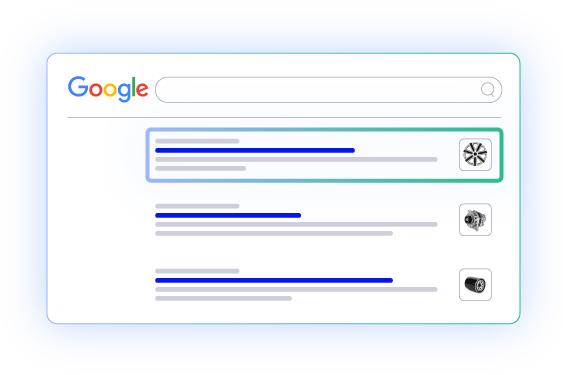The image features the Google logo prominently displayed at the top, with each letter distinctly colored: a blue G, red O, yellow O, blue G, green L, and a red E. Below the logo, there is an oval icon with a magnifying glass inside, which transitions from a blue to green gradient. Next to this, there are depictions of several lines and icons. 

Firstly, a sequence shows alternating gray and blue lines—starting with a gray line, then a blue line, followed by another series of gray lines. The second section includes an icon resembling machinery or an engine, again flanked by gray and blue lines in the same pattern. In the third section, another set of alternating gray and blue lines is displayed, accompanied by an icon of a cylinder. This cylinder appears to be mainly gray with hints of blue or green on the edges. The entire image is framed within a white window, creating a stark contrast with blue shadows outlining the edges.